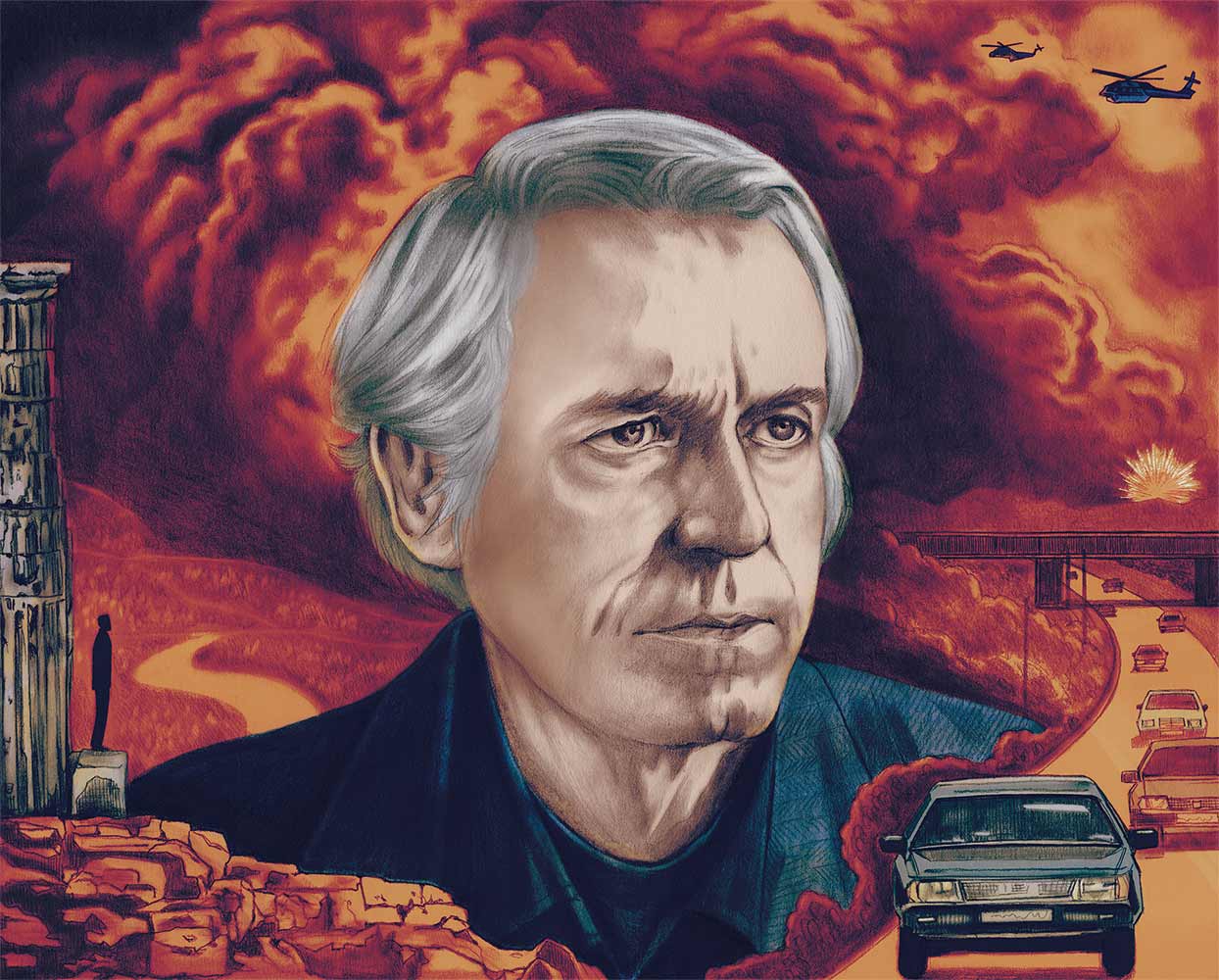The image is a detailed, artistic depiction resembling a chaotic movie poster. Dominating the center is a detailed drawing of a man with a light complexion, gray and black hair, and brown eyes. He is dressed in a black jacket and T-shirt, wearing a stern expression. Surrounding him are various dynamic elements: 

In the lower right corner, a blue sedan leads a convoy of six or seven cars of various colors, emerging from the center right towards the front of the picture on a highway. In the top right corner, two black silhouette helicopters fly against a dramatic backdrop of a yellow and red sky, indicating an explosion with red, orange, and black hues. Above them is a small image of the sun.

To the left, a marble arch rises from the bottom halfway up the frame, behind which stands the silhouette of a man on a pedestal. The lower left corner showcases rocks in shades of red, yellow, and brown. The overall scene is bright and clear, filled with natural light, giving an impression of a vivid and tumultuous narrative. The amalgamation of these elements—vehicles, helicopters, explosions, and the central figure—creates an image full of symbolic tension and drama, potentially alluding to a complex story or theme.